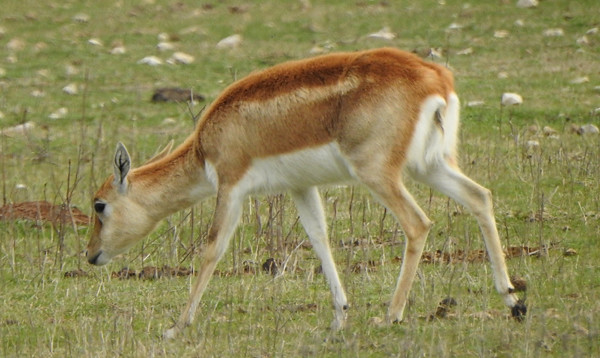The image captures a solitary, full-grown deer with a brown and white coat in an open, grassy field. The deer has its head down, seemingly sniffing or nibbling at the green and brown patchy grass. Surrounding the field are dirt patches, sprinkles of little white flowers, and a few scattered branches or bushes. In the background, there are various white and brown objects, possibly rocks or mushrooms, adding texture to the scene. The field is expansive, with no other animals or people in sight, suggesting it could be near a forest. The overall image has a landscape orientation, resembling the dimensions of a high-definition TV screen.